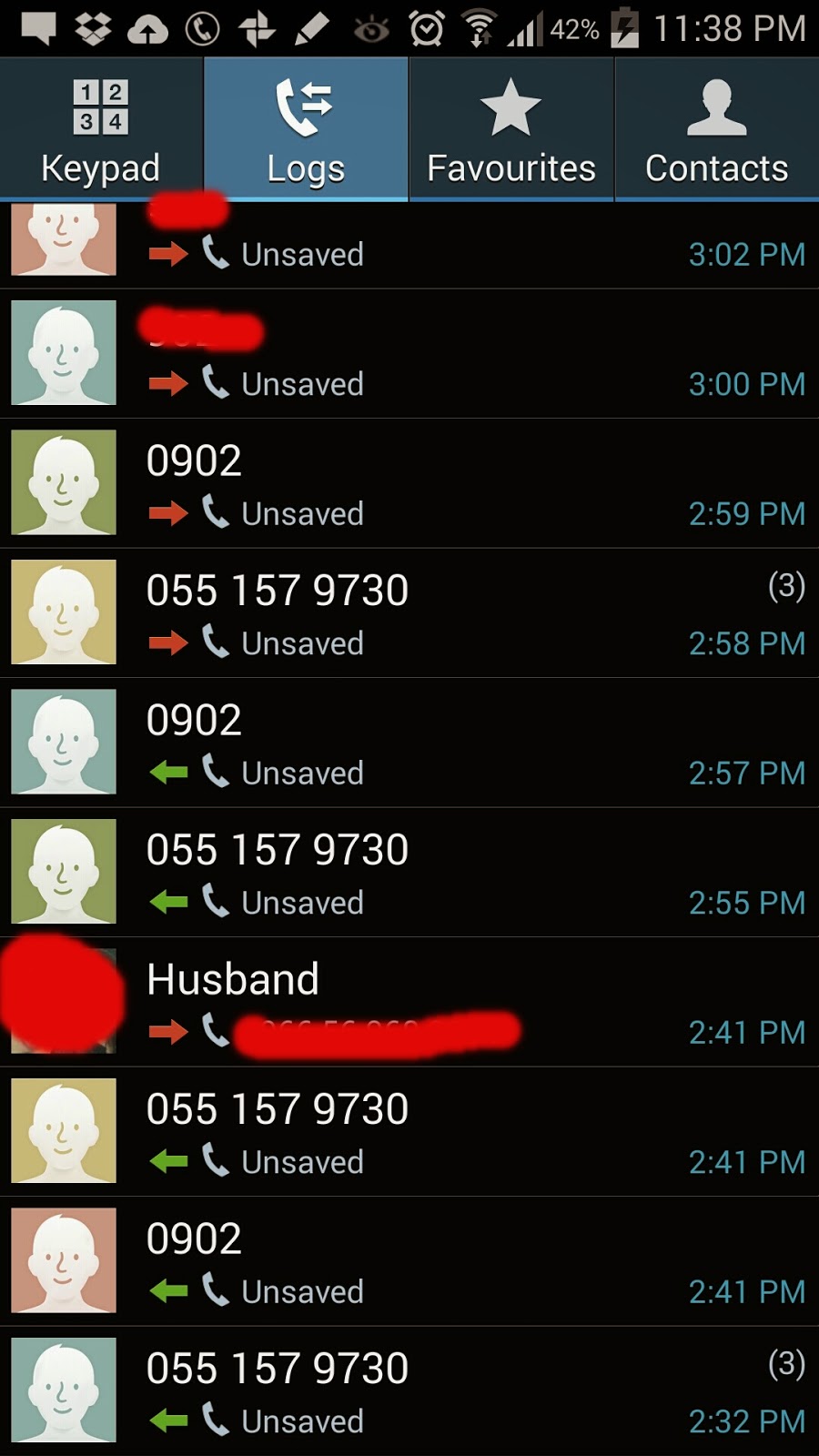A detailed screenshot of a cell phone's call log interface with a black background, displaying recent calls from various contacts. Vertically aligned icons in orange, blue, green, and yellow represent different callers on the left side of the screen. At the top, function buttons for the keypad, logs, favorites, and contacts are visible, marked with respective icons: a telephone with arrows for logs, a star for favorites, and a human figure for contacts. The top bar also features buttons to navigate to messages, phone calls, paint programs, and the alarm clock. Indicators show Wi-Fi connectivity, cell phone signal strength, and a battery level at 42%, with the current time being 11:38 PM.

The call log details include several unsaved calls listed at 3:02 PM, 3:00 PM, 2:59 PM, 2:58 PM, 2:57 PM, and 2:55 PM, along with a call from "Husband" at 2:41 PM. Additional entries show a call from the number 055-157-9730 at 2:41 PM and another unsaved call from the same number at 2:32 PM, as well as a call from the number 0902 at 2:41 PM. These comprehensive details provide a clear and organized view of recent phone activities.